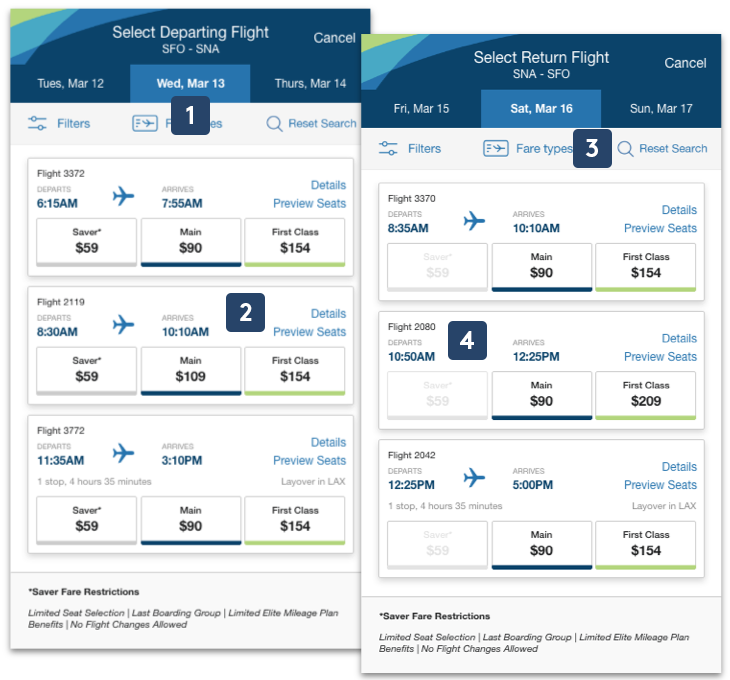This image contains two detailed flight selection screenshots. The left section is titled "Select Departing Flight" for a trip from SFO to SNA on Wednesday, March 13th. It showcases three flight options:

1. Flight 3372: Departs at 6:15 a.m. and arrives at 7:55 a.m., highlighted with a dark blue square with a white "1." Fare options include Saver for $59, Main for $90, and First Class for $154. Additional options include flight details and seat previews.
2. Flight 2119: Departs at 8:30 a.m. and arrives at 10:10 a.m., marked with a dark blue square with a "2." Fare options are Saver for $59, Main for $109, and First Class for $154.
3. Flight 3772: Departs at 11:35 a.m. and arrives at 3:10 p.m. after one stop and a 4-hour and 35-minute layover in LAX. Fare options include Saver for $59, Main for $90, and First Class for $154.

The saver fare includes restrictions such as limited seat selection, last boarding group, limited elite mileage plan benefits, and no flight changes allowed.

The right section is titled "Select Return Flight" for a trip from SNA to SFO on Saturday, March 16th. It features three flight options:

1. Flight 3370: Departs at 8:35 a.m. and arrives at 10:10 a.m., marked with a black square with a "3." The Saver fare is grayed out but listed as $59, Main fare is $90, and First Class is $154.
2. Flight 2080: Departs at 10:50 a.m. and arrives at 12:25 p.m., highlighted with a black square with a "4." The Saver fare is grayed out but listed as $59, Main fare is $90, and First Class is $209.
3. Flight 2042: Departs at 12:25 p.m. and arrives at 5:00 p.m. after one stop and a 4-hour and 35-minute layover in LAX. The Saver fare is grayed out but listed as $59, Main fare is $90, and First Class fare is $154.

All options list the same Saver fare restrictions as the departing flights.